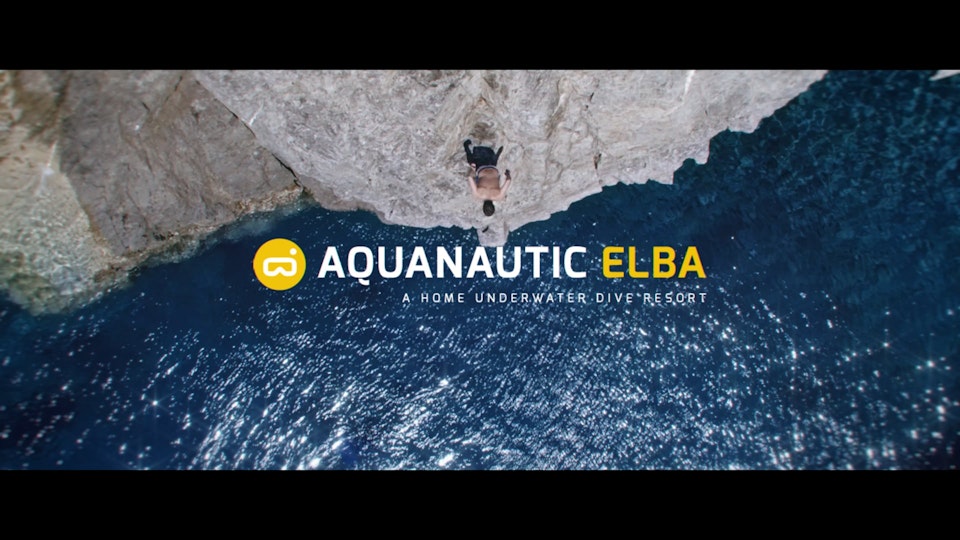The advertisement for Aquanautic Elba, a home underwater dive resort, presents a striking bird's-eye view of a diver poised on the edge of a rocky cliff. The diver, partially dressed in a diving suit and casting a shadow on the rocks beneath, appears ready to either put on or take off his gear. The image is split between the rugged gray and brown cliff at the top and the deep, dark blue water below, which glistens as it reflects the sunlight. The scene is framed by a thin black border at the top and a thicker one at the bottom. Central in the image is the brand's logo, depicting a pair of goggles with a dot above them. Across the blue water, the name "Aquanautic" is featured in white, followed by "Elba" in yellow-gold text. Beneath this, in smaller white font, reads "A Home Underwater Dive Resort." The overall effect is a captivating and inviting visual, enticing viewers with the thrill and mystery of underwater exploration.